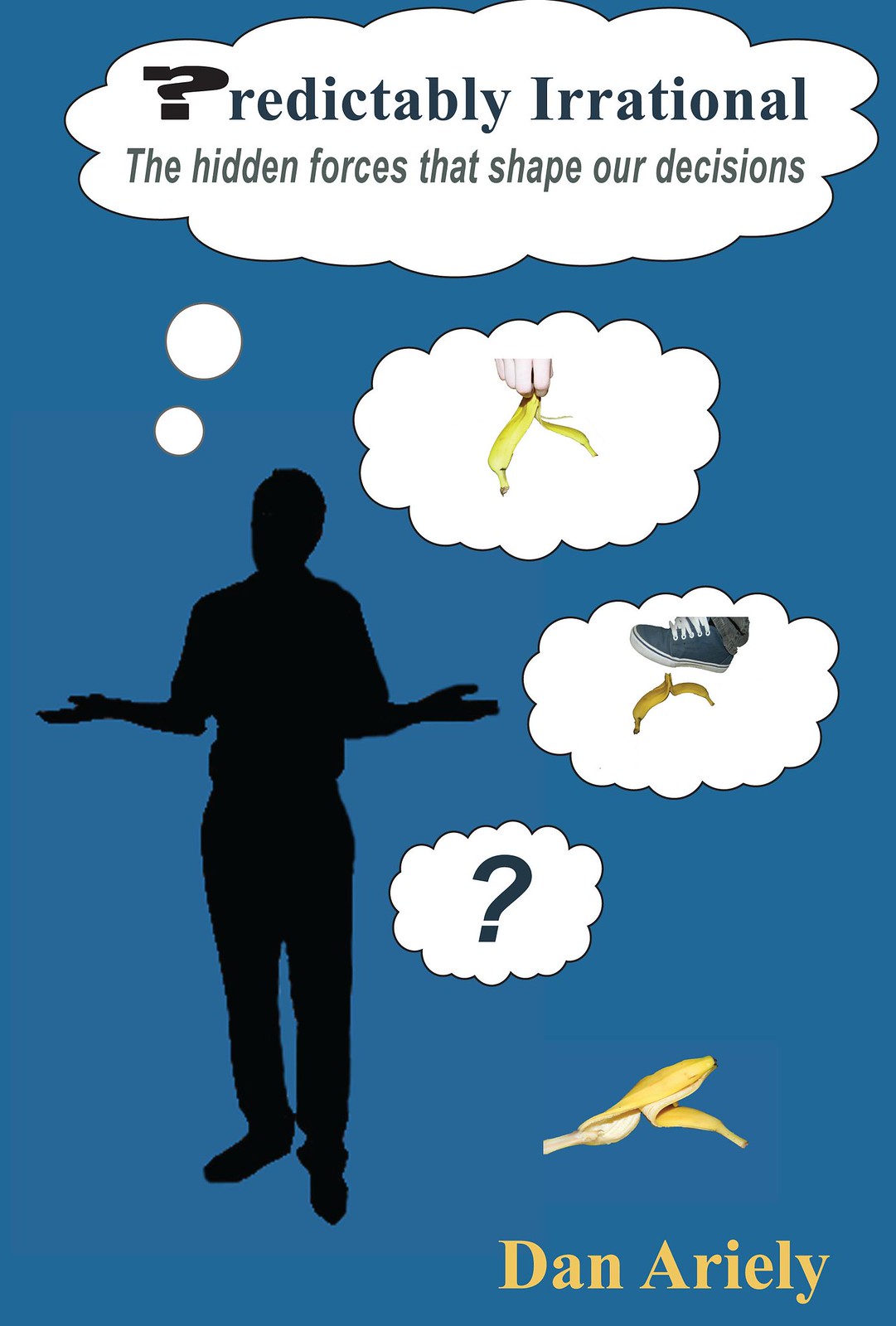The image features a solid blue background with the silhouette of a man, dressed in pants and a short-sleeved top, standing with his arms out in a questioning or shrugging posture. Above the man, a series of white thought bubbles rise. The first large bubble contains the text: "Predictably Irrational: The Hidden Forces That Shape Our Decisions." Below this bubble are three smaller ones. The first shows a white hand dropping a banana peel, the second depicts a foot in a blue tennis shoe with white laces about to step on the banana peel, and the third contains a large question mark. At the bottom of the image is a banana peel, with the name "Dan Ariely" written in yellow text to the bottom right. This design appears to be an elaborate depiction likely related to Dan Ariely's book, "Predictably Irrational."